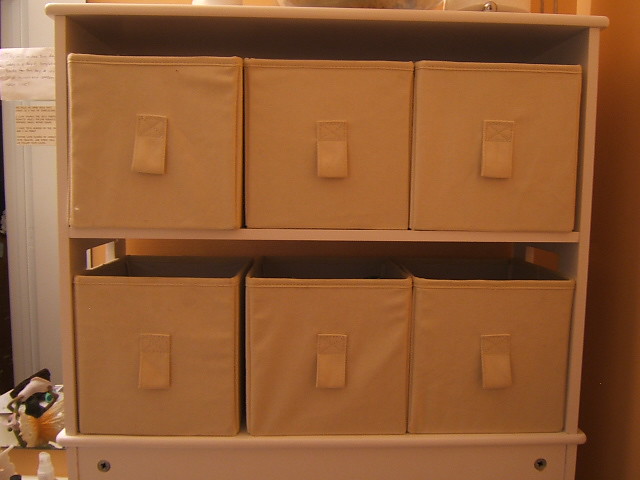The photograph showcases an indoor scene featuring a storage unit positioned against a white wall. The wall has two pieces of paper with writing on them, though they are too far away to be readable. Below the papers, on the ground, lies an object resembling a stuffed animal. The storage unit itself is designed to look like faux wood in a matching light brown, and consists of two shelves. Each shelf holds three square canvas boxes, making a total of six. These butterscotch brown canvas boxes feature thick tabs in the middle for easy handling. A white door is visible to the left side of the storage unit. Additionally, some trash can be seen near the shelf, adding a touch of realism to the scene. The overall arrangement suggests a practical setup, blending functionality with a touch of cozy aesthetics.